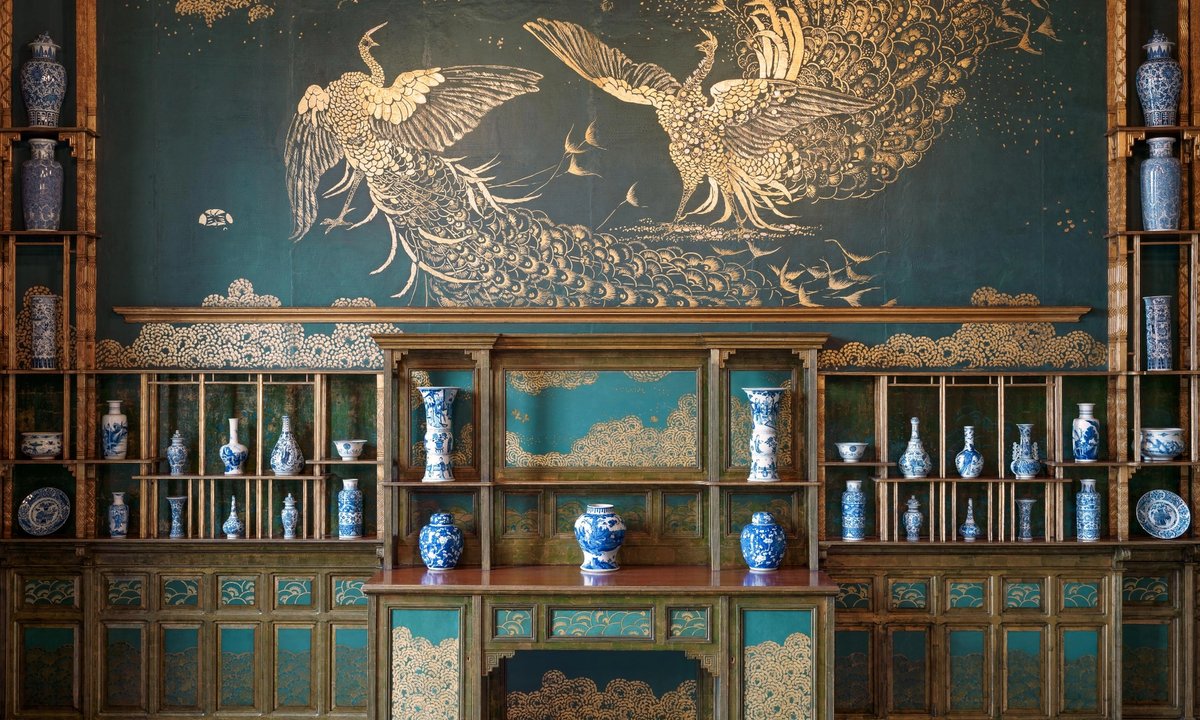The image depicts an elaborately decorated room with a distinct oriental ambiance. Dominating the scene is an extensive shelving unit of light brown, intricately built into the wall, featuring numerous cubby holes and shelves. Each cubby hole houses a porcelain vase adorned with traditional blue designs on a white background, creating a harmonious and cohesive aesthetic. Among these vases are also two plates, strategically placed at opposite ends of the arrangement. These meticulously displayed pieces of dishware draw the eye towards the centerpiece: a stunning mural showcasing two peacocks, intricately inlaid with gold against a backdrop of rich green and turquoise wallpaper. The mural, which appears integrated into the shelving unit, adds a majestic artistic touch to the room, emphasizing the room's luxurious and culturally rich design.